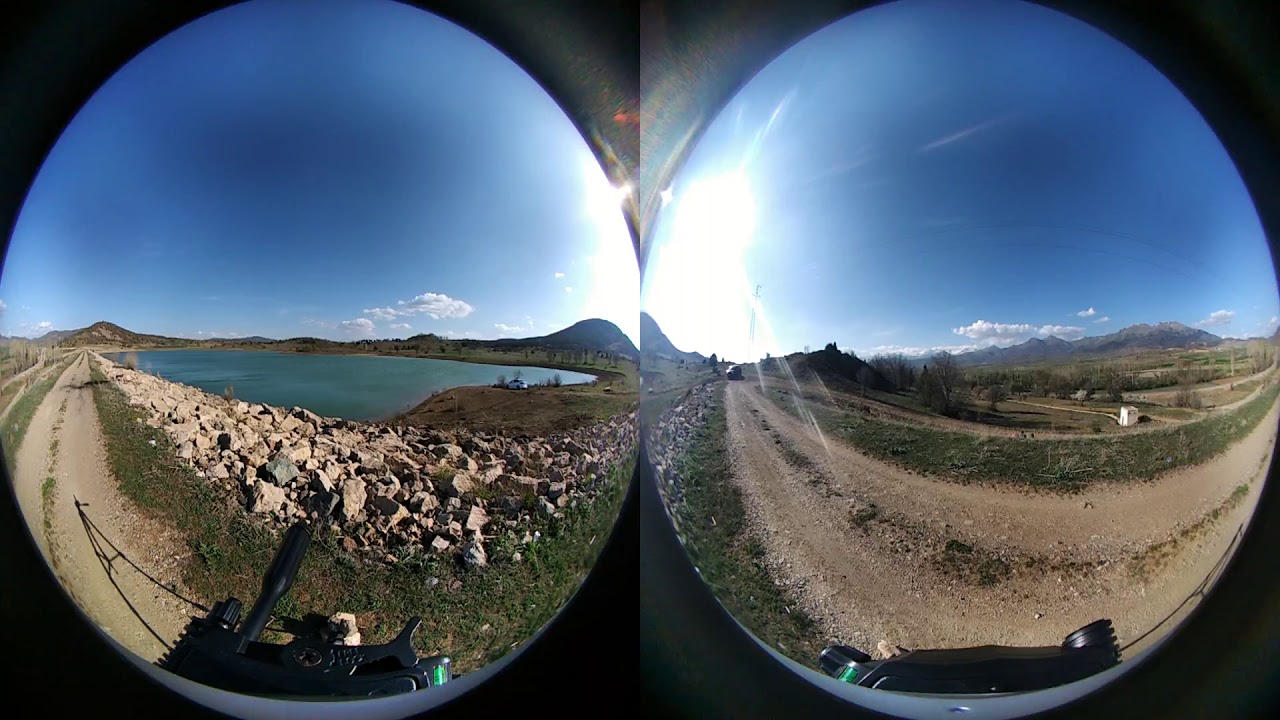This panoramic scene is captured using a dual fisheye lens setup, showcasing two interconnected images side-by-side. Both images are set against a backdrop of clear blue skies with minimal clouds, offering a bright and sunny view. The left image features a tranquil lake bordered by a rock wall, presumably for road protection. Foothills stand in the background, and a dirt trail meanders to the lake's grassy edge, where a parked car is visible. A camera setup atop a tripod, perhaps equipped with a selfie-stick handle, is discernible at the bottom edge of the frame. Moving to the right image, we see the continuation of the gravel road, still unpaved and bordered by grassy terrain. Mountains grace the background yet again, and new elements such as another dirt path and a small white structure, possibly a shed, come into view. This panoramic fusion creates a comprehensive vista that seamlessly merges two distinct yet complementary perspectives of this serene outdoor location.